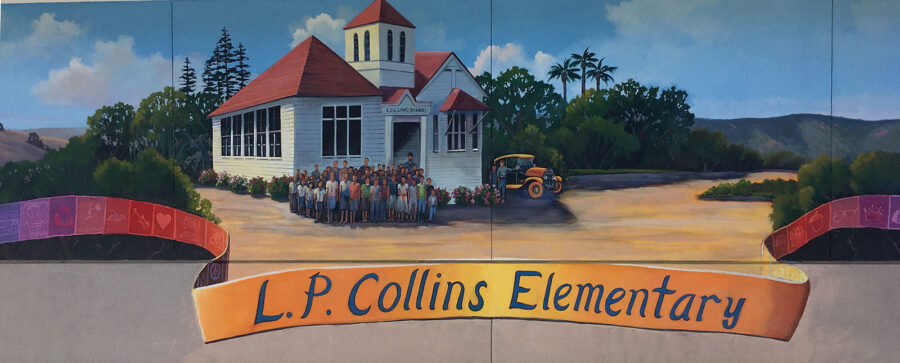This intricate mural depicts an old-fashioned schoolhouse with a distinctive red arched roof, separated into two sections on the left and right. The central section, adorned with white walls and a flat, cone-shaped roof, is punctuated by arched windows, giving it a church-like appearance. Highlighted by its tall, narrow windows with white frames, the structure has a nostalgic aura reminiscent of the 1920s or 30s. In the foreground, a tight-knit group of children gather as if posing for a photograph; many appear to wear gray or white shirts paired with gray shorts or skirts, although their features are blurred due to the artistic style.

To the right of the children, an old-fashioned yellow automobile, reminiscent of a Model T, adds to the historical ambiance. Two individuals stand nearby, enhancing the scene's vintage feel. Surrounding the schoolhouse, flowering bushes add bursts of color, while the backdrop of tall pine and palm trees further enriches the scenery. Above, the sky transitions from a clear blue in the center to gray cloud-filled edges.

Across the image, a banner with blue letters spelling "L.P. Collins Elementary" stretches from left to right, decorated with alternating red, purple, and pink squares. The natural lighting and detailed portrayal suggest this mural, possibly adorning an outdoor wall, beautifully captures the essence of a bygone era while celebrating the heritage of the school.